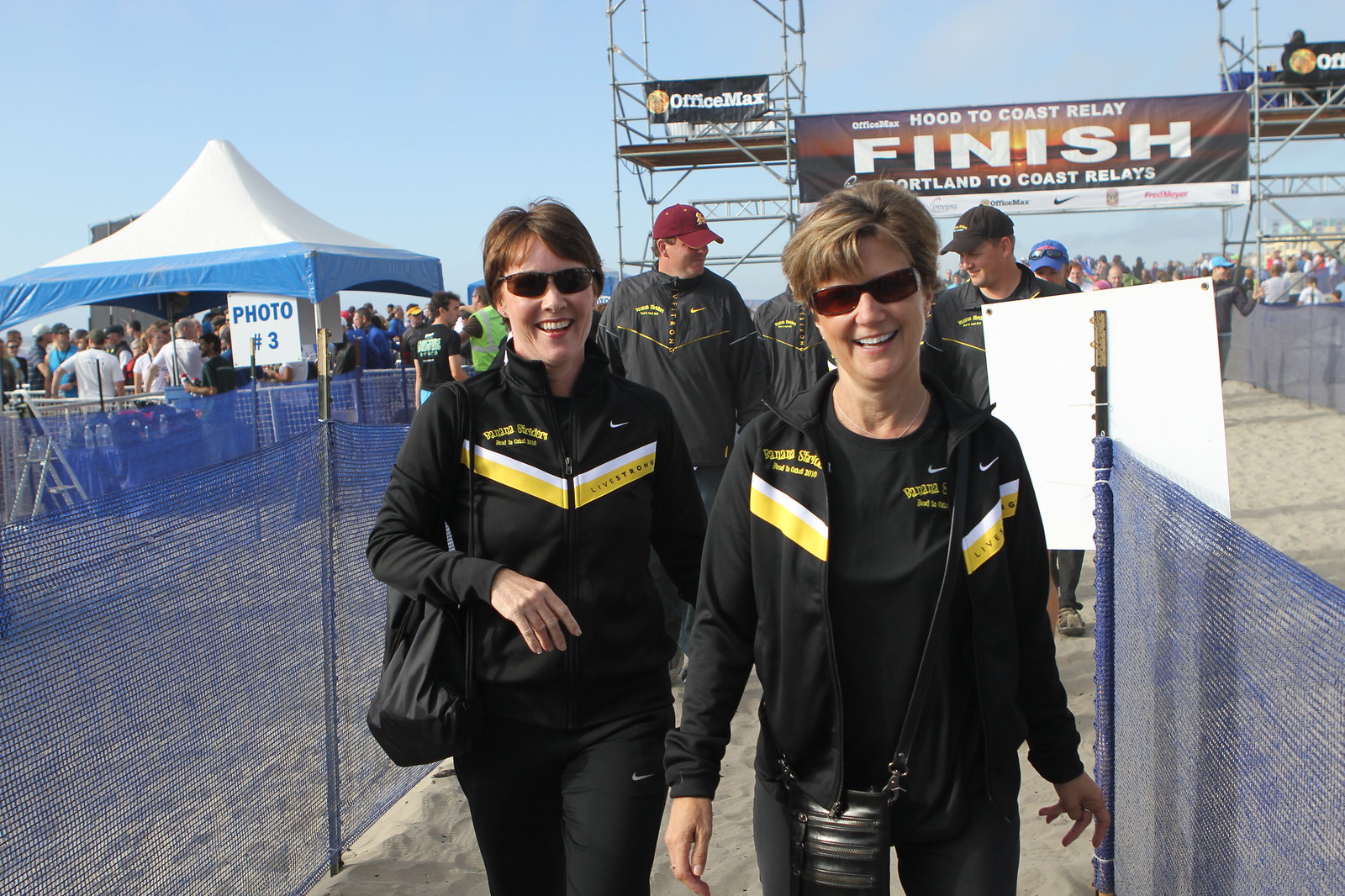The image depicts a vibrant and bustling scene at the finish line of the Hood to Coast Relay race. Two women, both brunette and smiling, stand prominently at the forefront. The woman on the right wears boxy sunglasses, while the one on the left sports more oval-shaped eyewear. Both are dressed in matching black Nike jackets adorned with white and yellow "LiveStrong" logos, complemented by black workout pants and purses slung over their right shoulders. Their outfits are partially zipped, with the woman on the right having her jacket open. They walk on a path of white or tan sand flanked by blue mesh fencing, guiding participants toward the finish line.

In the background, a silver bracket structure supports banners that read "Hood to Coast Relay Finish" and "Portland to Coast Relays." Behind the women, multiple participants clad in similar Nike attire, including maroon, black, and blue hats, bolster the sense of camaraderie at the event. A white and blue tent marked "Photo Number Three" is set up on the left, with clusters of people mingling beneath. The sky above is a clear blue, illuminated by the yellow sun, suggesting an outdoor, coastal setting. Off to the right, there’s a white sign—its text obscured as it faces away—beneath which more individuals gather, hinting at the popularity and significance of this relay race.